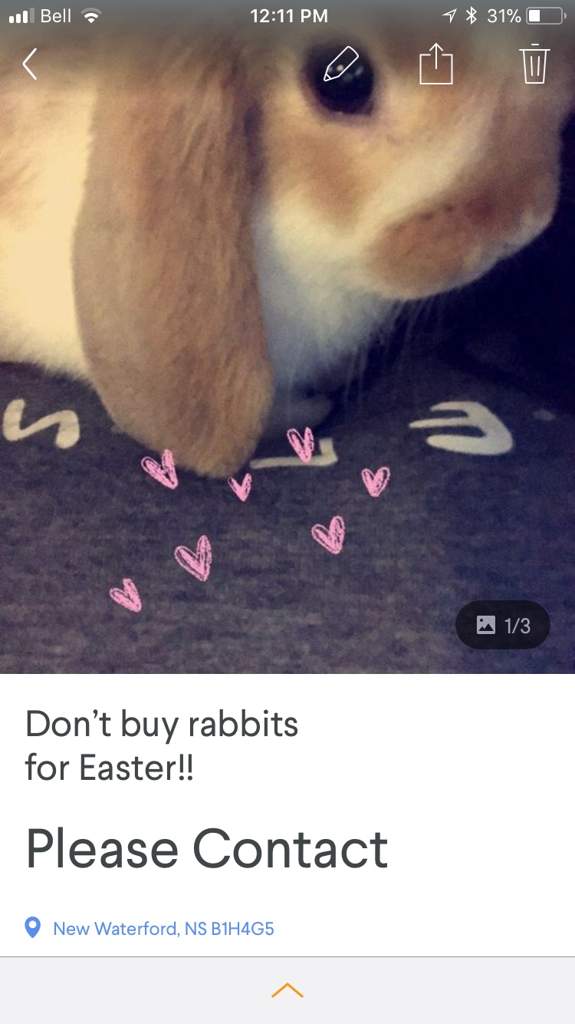The image showcases a cute rabbit illustration adorned with small hearts scattered around it. The top part of the image includes several elements indicative of a screenshot from an iPhone device: the time displayed is 12:11, and in the upper left corner, icons for a Wi-Fi signal labeled "Bell," a Bluetooth connection, and a battery life indicator showing 31% are visible. Additionally, within the middle section of the image, there is a label that reads "1 of 3" with an accompanying icon. Below the main illustration, text urges viewers not to buy rabbits for Easter, with a plea to "please contact." A notification displaying "Blue New Waterford, NS B1H 4G5" is also present. The bottom part of the image features a gray section with an orange upward-pointing arrow. 

Overall, the image integrates a strong message about responsible pet ownership within a brightly decorated and functional smartphone interface.